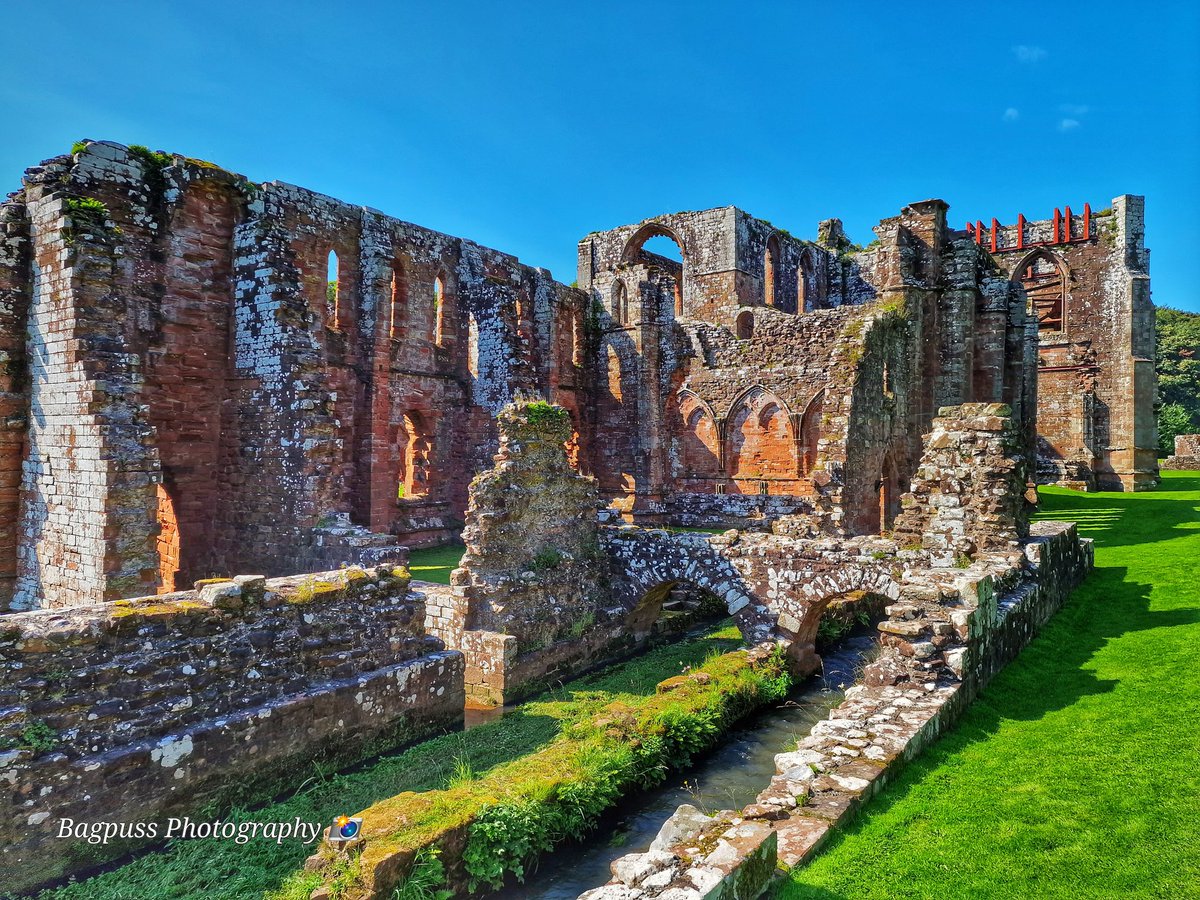This photograph, taken by Bagpuss Photography and marked with their logo in the bottom left corner, captures the striking remnants of an ancient, majestic structure that resembles a castle or palace. The edifice, made predominantly of reddish-brown stones with fading remnants of white paint, stands in significant ruins. Its once grandiose features, such as arched doorways, turret-like windows, and multi-story walls, are now interspersed with crumbling bricks and covered in lichen. Despite its dilapidated state, many of the walls remain intact, conveying a sense of historical grandeur.

A serene stretch of water meanders through the middle of the scene, spanned by a partially intact bridge. Surrounding the ruins, the landscape is dotted with lush, green grass and bordered by a dense forest visible in the background. The vivid blue sky, adorned with a few wispy clouds in the top right corner, highlights the picturesque beauty of the setting, which is bathed in the light of a bright, sunny day.